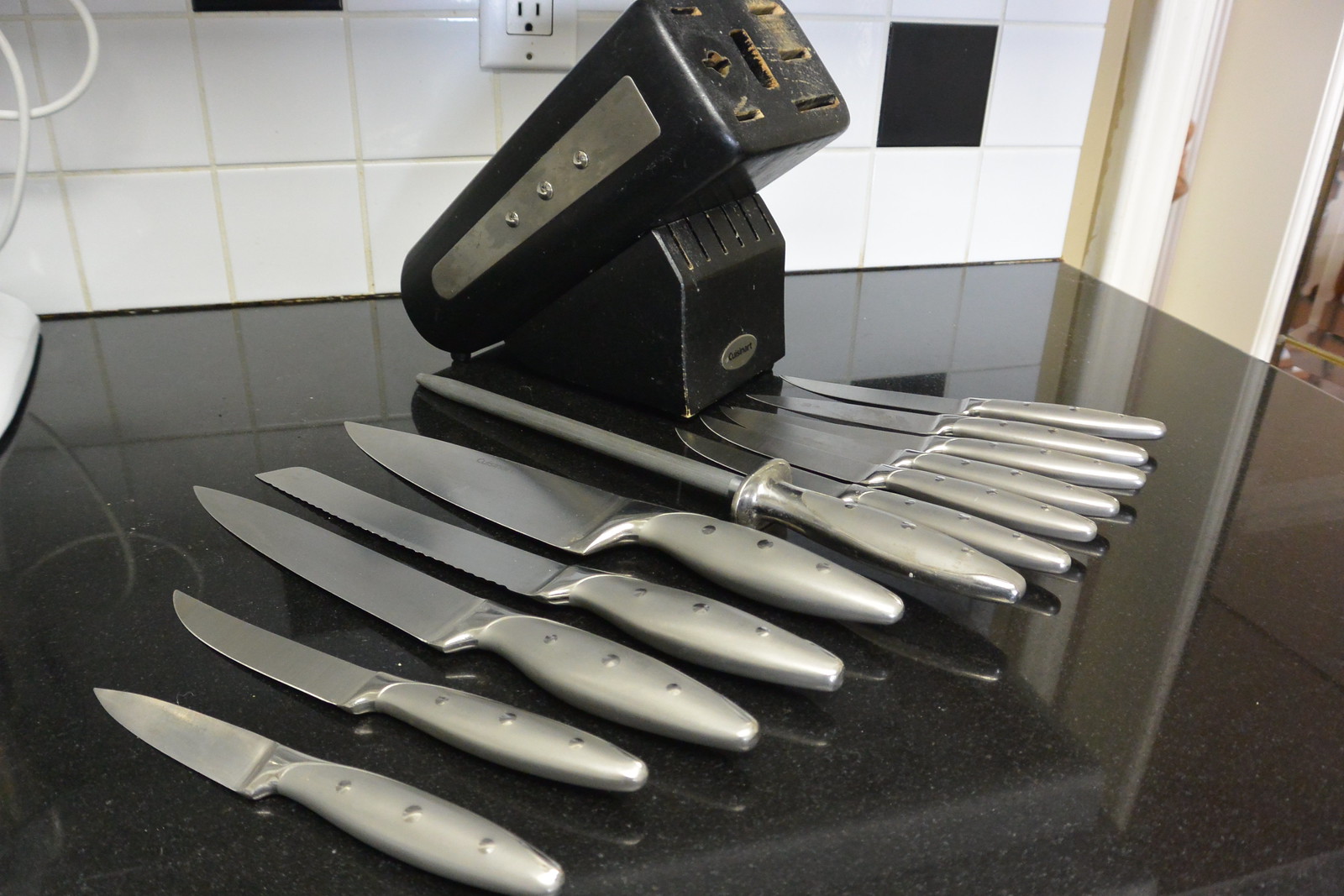This photograph captures a well-used kitchen scene showcasing an array of approximately 15 silver stainless steel knives of varying shapes and sizes. The knives are meticulously laid out diagonally from the lower left to the upper right on a shiny, smooth black countertop, possibly made of granite or marble. On the left side of the image, the larger knives such as chef and butcher knives are prominently displayed, whereas the smaller paring and steak knives are positioned towards the right. In the center among the knives lies a knife sharpener. At the tips of the smaller knives, a black, slightly rusty knife holder with individual slots for each knife sits on the countertop. The background features a white tiled backsplash interspersed with a few black tiles for a touch of character. On the far right side, a white wall and part of a doorway leading into another room are visible. Additionally, a portion of an electrical outlet peeks out from the backdrop, completing this detailed composition of a practical kitchen space.